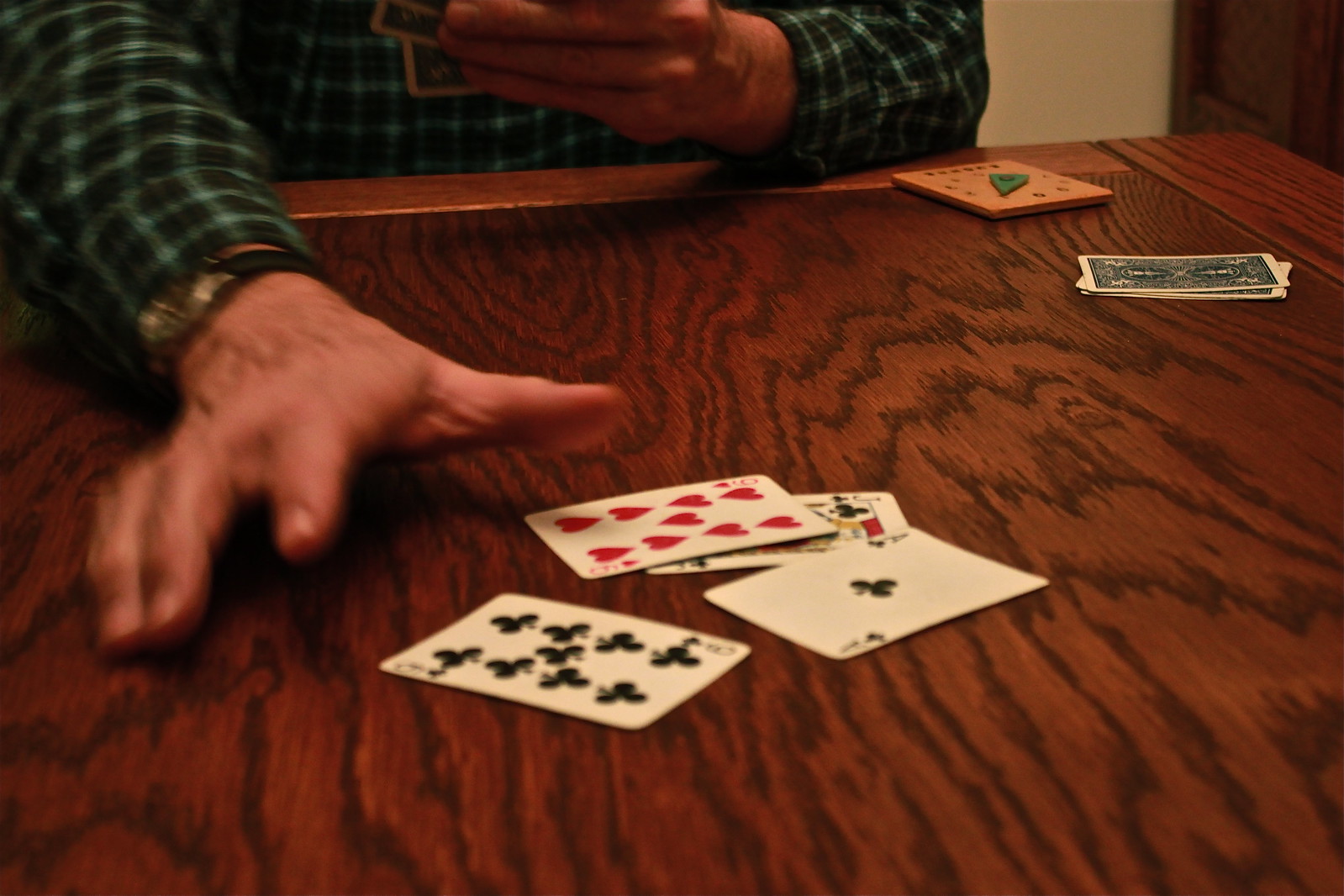In this photograph, a person is seated at a wooden table, engrossed in playing cards. The individual, identifiable by the slightly hairy and rough-looking wrist, is wearing a dark gray or forest green plaid shirt accented with lighter green stripes. A black wristwatch adorns the person's left wrist. This hand is positioned to reach for some cards lying on the medium brown, wood grain table. The table's surface reveals distinct black wood grain patterns, adding texture to the scene.

The right hand holds a set of cards with a distinctive white strip around the edges and a blue and white design. Various cards are scattered face-up on the table, including some from the club suit and at least one from the heart suit. Located near the person's elbow on the table is a square brown object topped with a green item, with additional cards nearby. The backdrop includes a sliver of a white wall and what seems to be another wooden surface, partially visible behind the person's elbow, providing context to the setting.